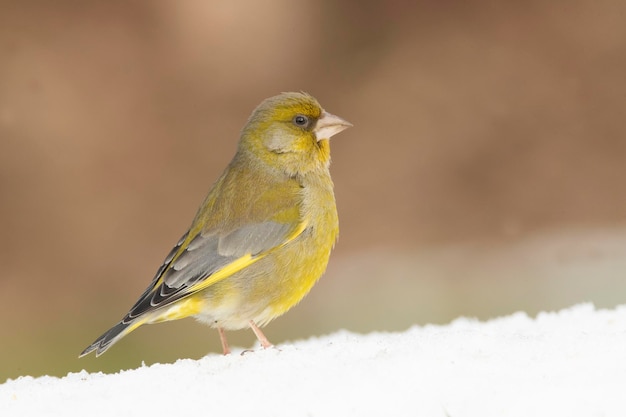In this detailed image, we observe a small, delicate bird resembling a sparrow, prominently featuring yellow and gray hues. The bird stands on a granular, white surface that gently inclines upwards to the right, giving the impression of traversing a light snow blanket. It is captured in a side view, oriented towards the right, with notable yellow on its head, breast, and belly. The wings and tail exhibit a mix of gray and black, with the most vibrant yellow found beneath the tail and at the edges of the wings. The bird also has striking black eyes, a light gray cheek, and a very pale beige beak. The background of the image is blurred and predominantly showcases varying shades of brown, creating a contrast that highlights the bird’s vibrant coloration.